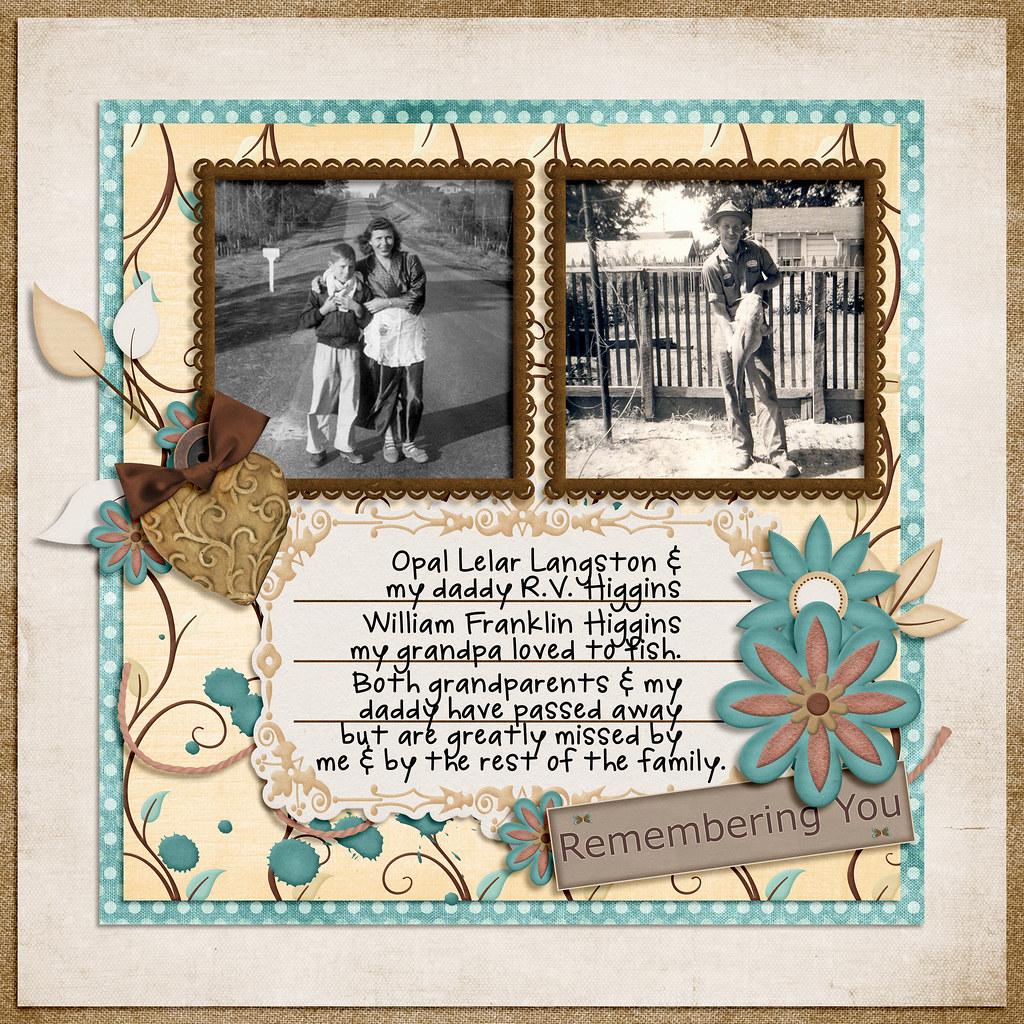This scrapbook page, framed by a brown border, features two side-by-side black and white photos set against a decorative background adorned with flowers and hearts. On the left, a young boy with short hair, wearing khaki pants and possibly a backpack, stands on a road beside a white mailbox, embraced by a woman with brown hair, dressed in either an apron or a silken bathrobe. Surrounding them are trees flanking the road. The right photo captures an older man, sporting a fedora hat and a polo shirt typical of a mechanic, proudly holding a large catfish. He stands in front of a fence, with a small house and more trees visible in the background. Below the photos, text memorializes family members with the words: "Opal Theiler Langston and my daddy R.V. Higgins. William Franklin Higgins, my grandpa loved to fish. Both grandparents and my daddy have passed away but are greatly missed by me and the rest of the family." A smaller text box in the bottom right corner reads "Remembering you."